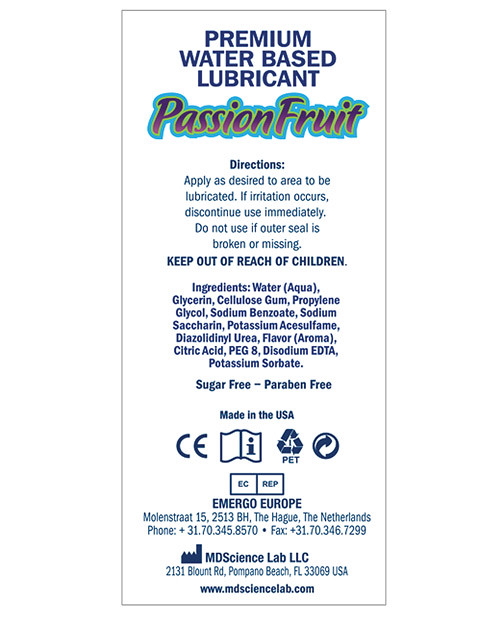The image features a label for a premium water-based lubricant, prominently branded with "Passion Fruit" in eye-catching purple letters outlined in blue. Beneath the product name, detailed directions are provided: "Apply as desired to the area to be lubricated. If irritation occurs, discontinue use immediately. Do not use if the outer seal is broken or missing. Keep out of reach of children."

Further along the label, a list of ingredients is outlined: water, glycerin, cellulose gum, propylene glycol, sodium benzoate, sodium saccharin, potassium, flavor and aroma, citric acid, disodium, and potassium sorbate. Noteworthy product features are also highlighted, including being sugar-free, paraben-free, and made in the USA.

The label also contains four distinct symbols at the bottom: the recycling symbol, the "CE" mark, a book with the letter "i" indicating informational instructions, and a circular symbol with an arrow, suggesting recyclability or environmental friendliness.